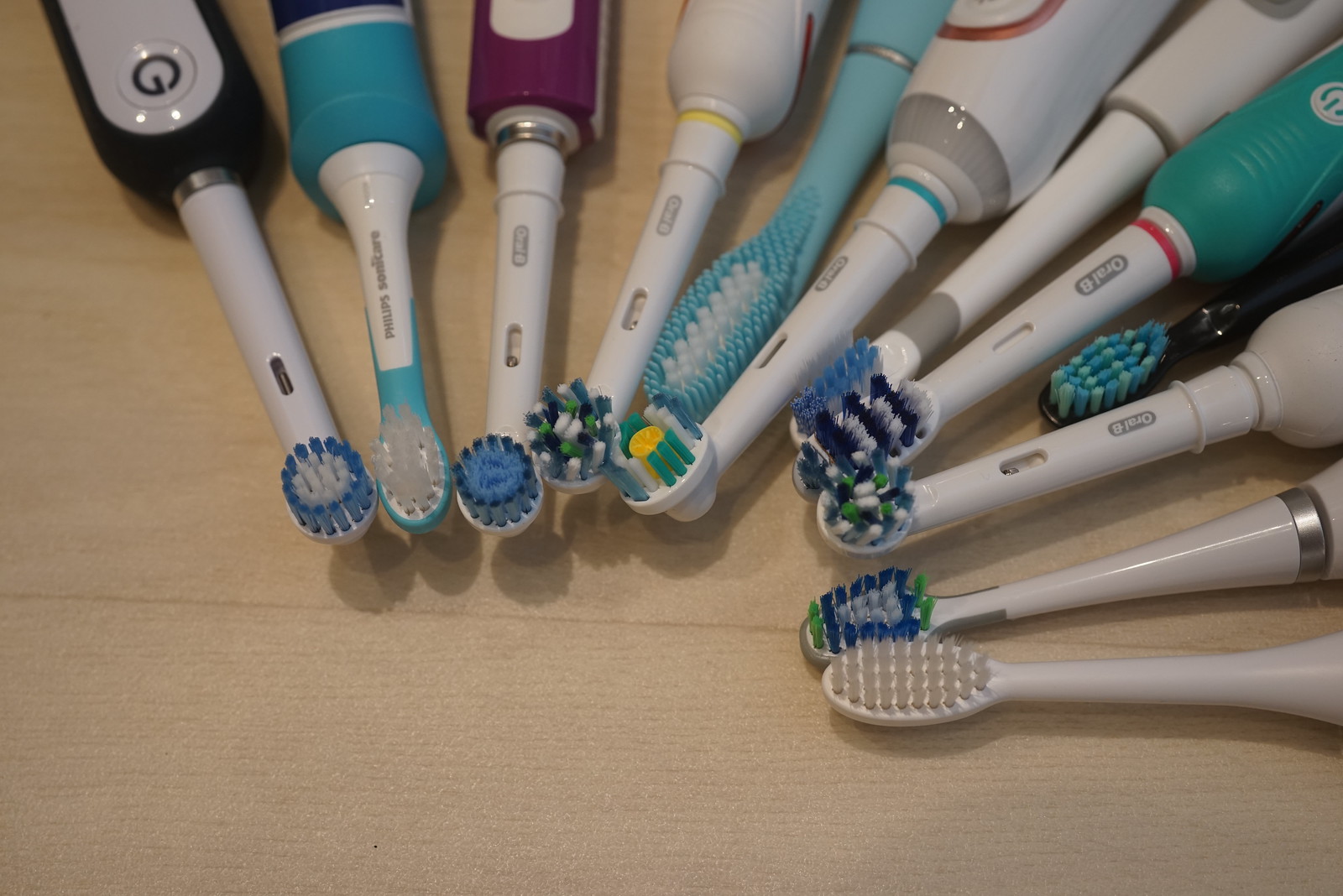This is a close-up photograph of various types of toothbrushes, primarily electric, arranged in a circular fashion with the bristles meeting in the center. The toothbrushes differ significantly in style, color, and design. The collection includes both standard and electric toothbrushes, with some featuring bristles in round or oval shapes and others having more traditional, elongated bristle layouts. The toothbrushes are arrayed on a cream-colored surface, likely a table.

Some toothbrushes have multicolored bristles, while others have bristles that are uniform in color. One particular toothbrush features only rubber bristles, with larger ones on the inside and smaller ones on the outside. The bristles themselves vary in height and protrusion. The toothbrush handles are predominantly white, contrasted by the colorful bases in shades of black, blue, purple, yellow, and clear. Notable brands like Oral-B are visible among the assortment. Overall, the image captures a diverse and visually striking display of dental hygiene tools.